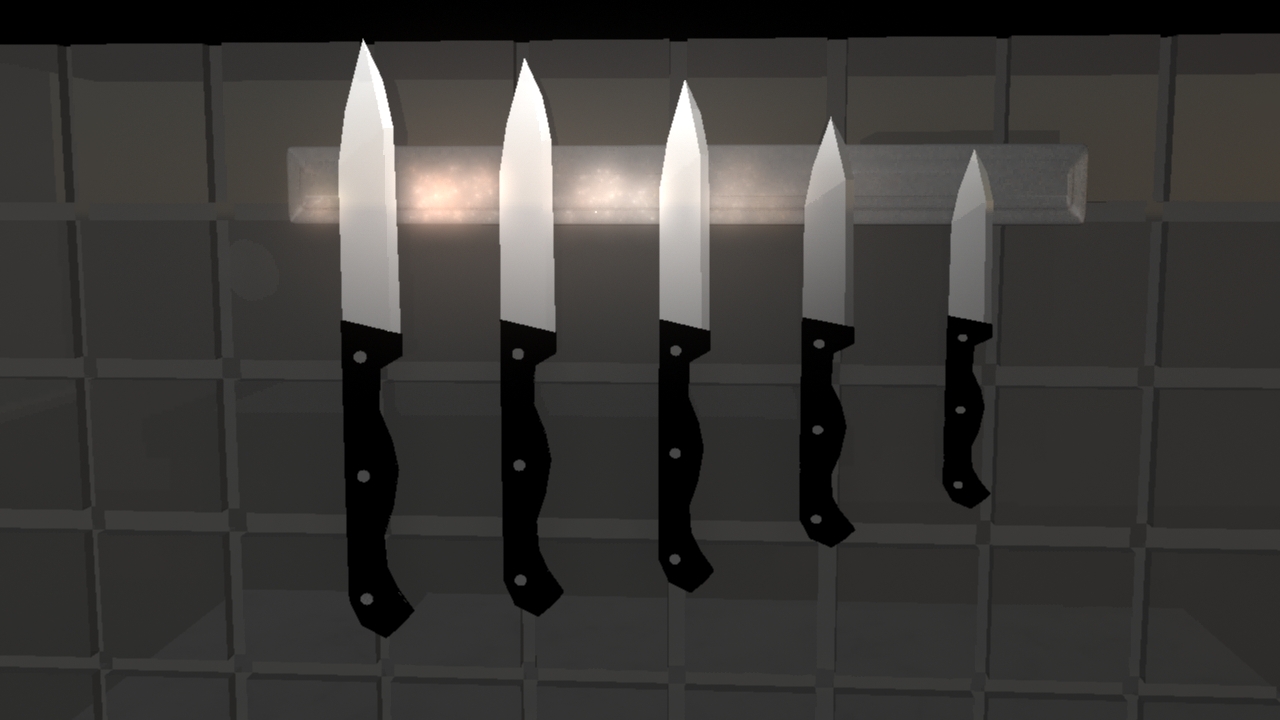This image features a set of five knives neatly arranged on what appears to be a metallic magnetic knife rack, mounted on a background of dark gray, square-patterned tiles. The knives, identical in style, vary in size from largest on the far left to smallest on the far right, creating a descending order. Each knife boasts a silver blade and a jet-black handle, crafted with three metal rivets securing the handle to the knife. The magnetic rack, silver-hued, securely holds the knives by their blades, likely in a kitchen setting. The overall configuration and consistent aesthetic of the knives suggest they belong to the same set, perfectly aligned against the grid-like, dark gray tiled wall.